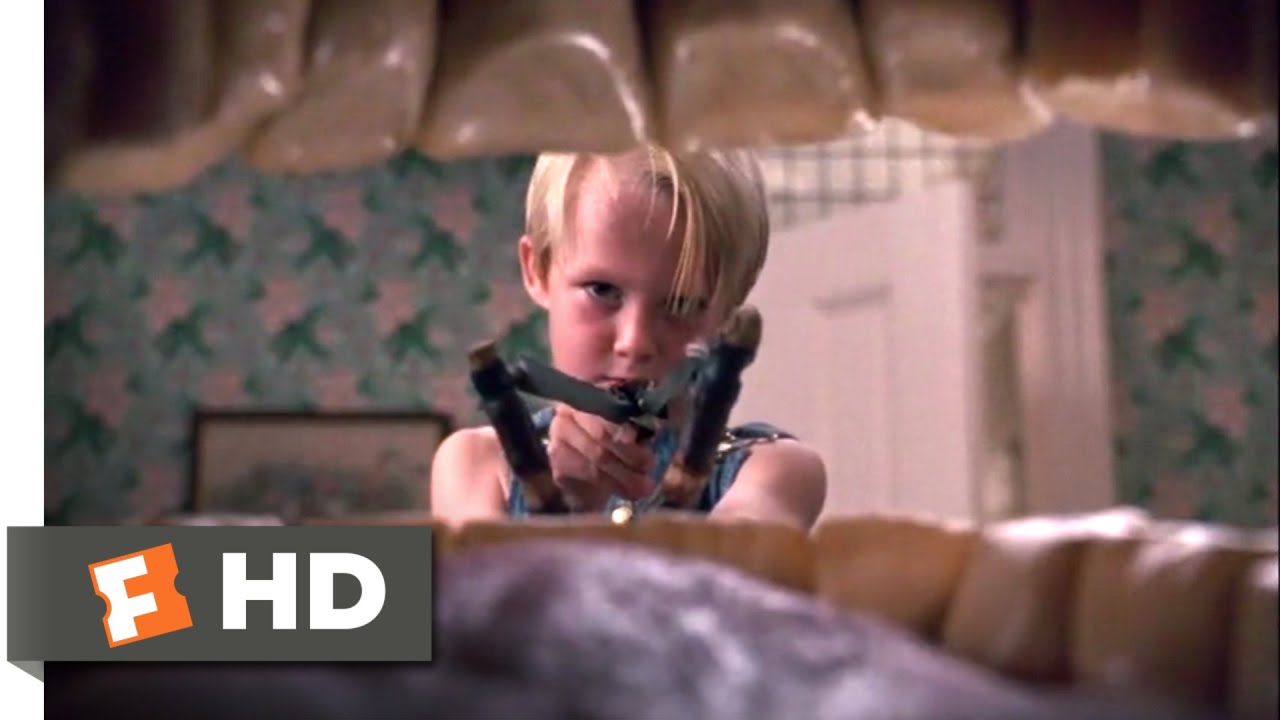This detailed image composition, likely taken from a still in one of the Dennis the Menace movies, prominently features a young boy, approximately eight or nine years old, with straight blonde hair parted to his right. His hair falls to his left as he scowls mischievously. The boy is firmly gripping a wooden slingshot, shaped like a V, and tugging back its black leather band, seemingly ready to launch a projectile. Notably, the viewer's perspective is from inside an open mouth, revealing the upper and lower teeth along with the tip of a tongue in the foreground. In the blurred background, floral wallpaper with pink flowers and dark green leaves can be seen, alongside a partially open white door. A gray rectangle with an orange square and a white "F" logo for Fandango is visible in the bottom right corner, marked with "HD" to indicate high definition.